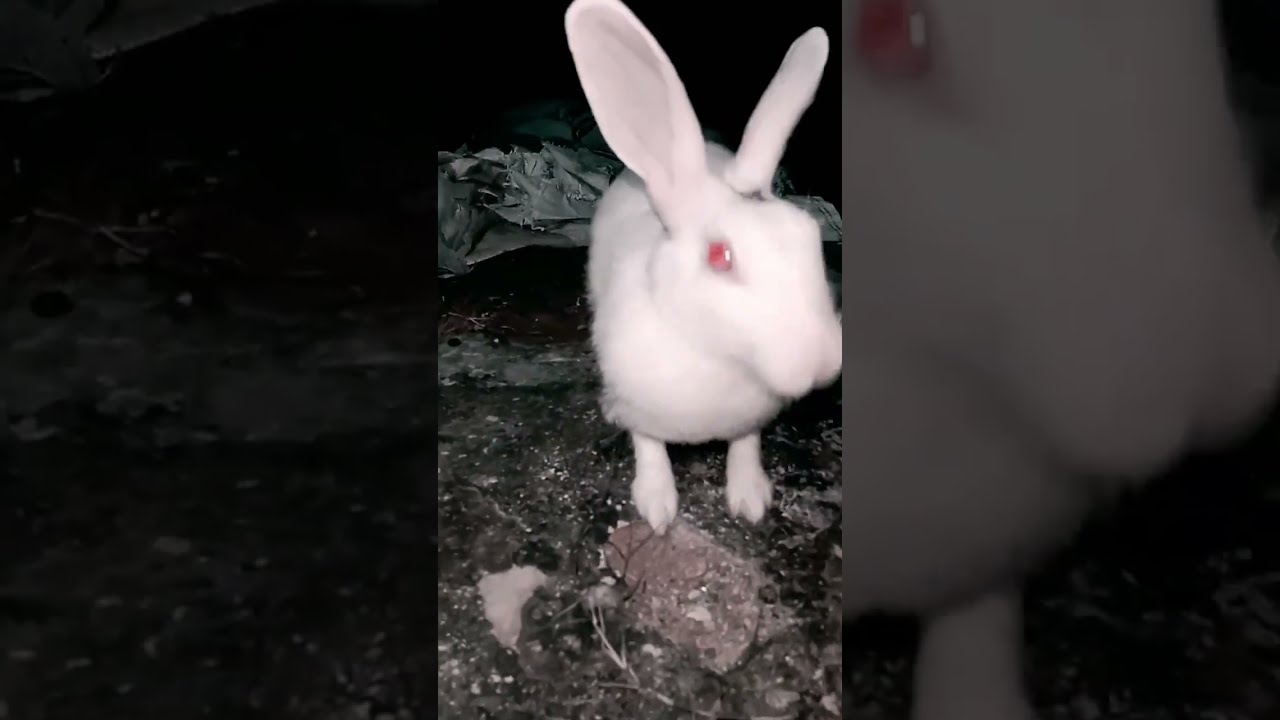The image is a horizontally rectangular composite consisting of three sections: a left vertical rectangle, a middle vertical rectangle, and a right vertical rectangle. The left and right sections are dark and unclear, blending into the obscured background of the nighttime outdoor scene. The middle section is better lit and focuses on a white rabbit standing on what appears to be an outdoor stone surface. The rabbit is facing forward and slightly to the right, with its long ears extending straight upward. Its right eye, which is a pale red color, is visible and appears to be looking slightly to its left. The rabbit's front paws are on a rock, and behind it, there is indistinct debris that could be trash or natural elements like leaves and branches. The right section provides a zoomed-in and blurry close-up of the rabbit's head, showing the same red eye and part of its face, along with a bit of the ground or rock it stands on. The blurred details and darker tones create a muted, almost transparent effect around the central clearer image.